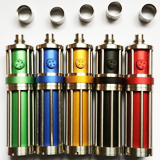The image depicts five cylindrical objects arranged in a row, side by side, within a square frame that is predominantly white. These objects are primarily characterized by their uniform metallic design, and they are distinguished by their colors, which from left to right are green, blue, yellow, black, and red. Each cylindrical object features a metal ring at the bottom, two additional rings in the middle, and a circular disc at the top, all of which contribute to their sleek metallic sheen. Above these cylinders, there are five small round metal components aligned horizontally. The specific function of these objects is unclear due to the image's small size and lack of detail. The lighting is bright, suggesting that this may be a promotional photograph.